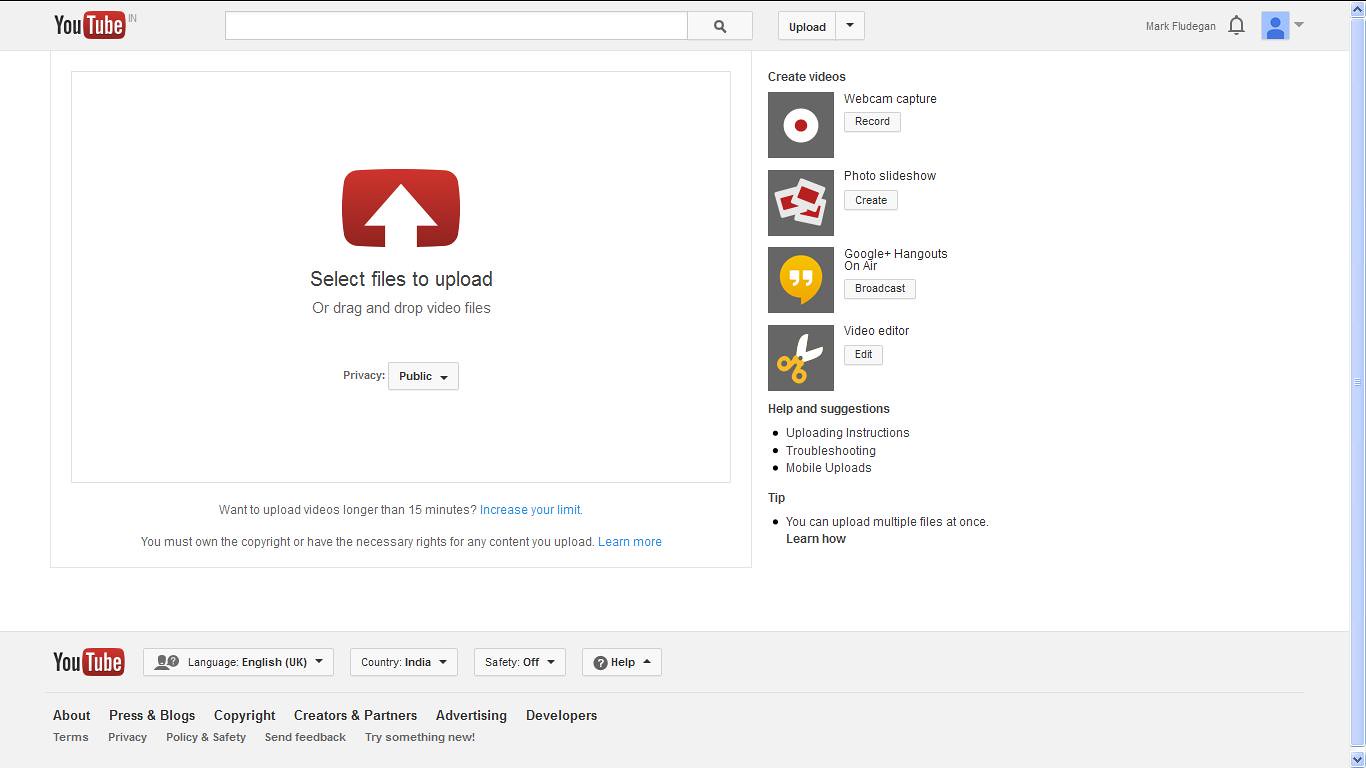The image depicts a screenshot of a YouTube upload page, featuring a predominantly white or off-white background. In the top left corner, the recognizable YouTube logo is prominently displayed. Across the top is a search bar, and in the top right corner, there is an icon resembling a blue person outline alongside a bell notification symbol.

The main section of the page has a central prompt that says "Select files to upload." This area is highlighted by an arrow graphic inside a red triangle. Additionally, it mentions, "or drag and drop video files," indicating alternative upload options. Adjacent to this, there are various icons and options including, but not limited to, webcam capture, photo slideshow, and creating videos from different types of files.

Further down, a banner of off-white hue contains multiple navigational links. It repeats the YouTube name and specifies the language as English. This banner offers links titled Help, About, Press & Blogs, Copyright, Creators & Partners, Advertisers, Developers, Terms, Privacy Policy, and Safety. A vertical scroll bar is visible on the right side, enabling users to browse the page content.